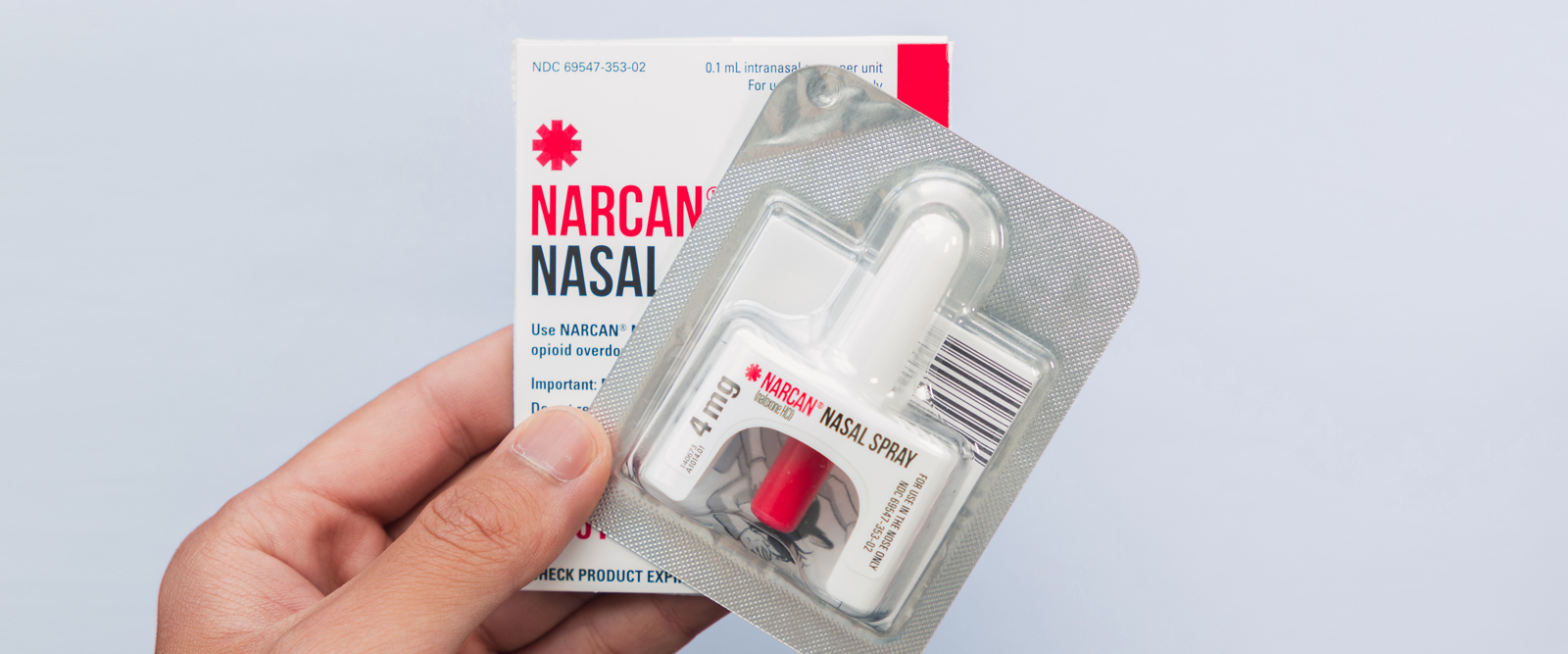The image features a well-lit, stock photo-quality depiction of a Narcan nasal spray package, set against a grayish-white background. The focal point of the image is a hand, emerging from the lower left corner, gripping the Narcan nasal spray box and its vacuum-sealed silver pouch. The hand appears to be female. The Narcan nasal spray, which is used to reverse opioid overdoses, is displayed prominently. The box features a red circular logo and blue text, including "4MG" and "Narcan Nasal Spray." The spray itself, visible inside its clear plastic packaging, is white with a small red section at the bottom and a protruding nose applicator. The image is designed to clearly showcase the product, possibly for advertising or an online listing.